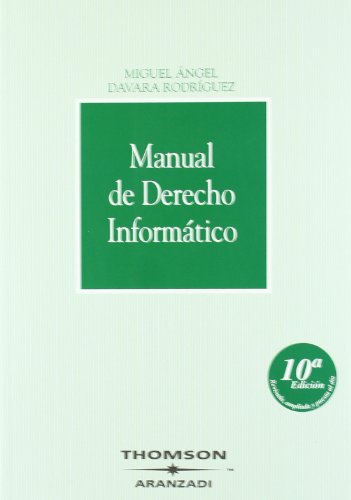The cover of this textbook, titled "Manual de Derecho Informático," is predominantly mint green with a bright green square framing the title in the center. The authors' names, Miguel Ángel and Davara Rodriguez, are positioned above this square box. Below the box and slightly to the right, a round circle marks the book as the 10th edition. The text on the cover, including the title and edition, is in white lettering. At the very bottom of the cover, the publisher's information is displayed in a distinct format: "Thomson" at the top, a star with outstretched wings in the middle, and "Aranzati" below. The overall design features a harmonious green color scheme with subtle variations to highlight different text elements.